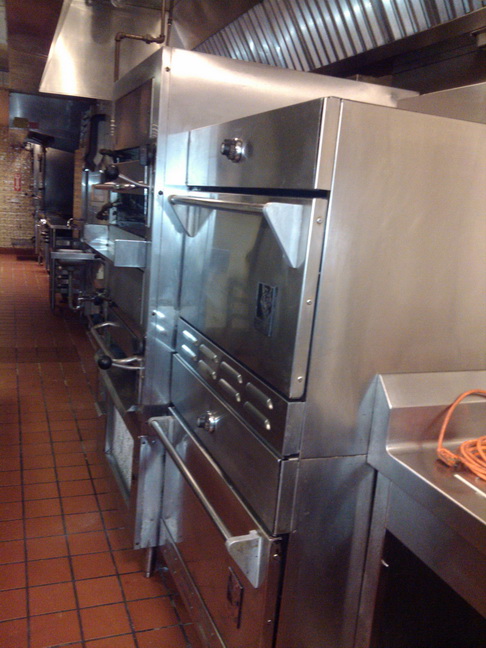The photograph captures a comprehensive view of an industrial, galley-style kitchen, likely within a bustling restaurant or perhaps an institutional setting. The floor is uniformly tiled in square, terracotta-colored tiles, radiating an earthy, reddish hue. The perspective of the image draws the eye down the length of the kitchen, with appliances arranged methodically along both sides. The nearest appliance is a sizable stainless steel oven, complete with a pull-down round handle. Flanking it is another similarly imposing oven, indicating a double-decker setup with one oven atop the other. Adjacent, and perhaps even taller, are more stainless steel appliances, which might include additional ovens or even salamanders, extending further into the depth of the galley. A sturdy prep table with a distinctly orange rope lies to the right, suggesting readiness for culinary tasks. The distant background is defined by a cream-colored brick wall, adding a subtle contrast to the metallic sheen of the appliances. This meticulously organized kitchen space, filled with industrial-sized stainless steel equipment, stands as the epitome of a professional culinary environment.